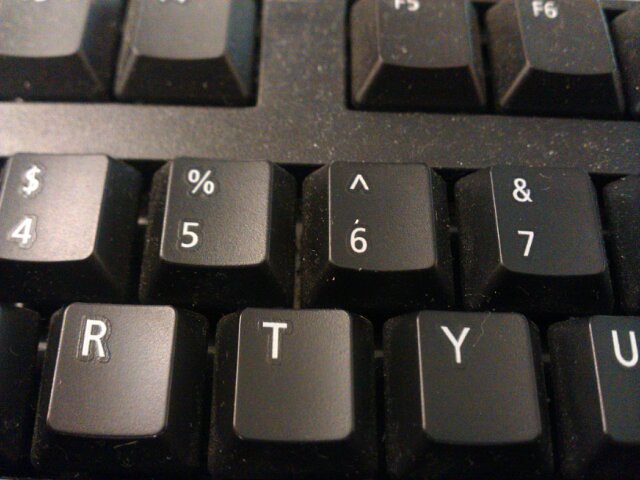This image is an extreme close-up of a dusty American QWERTY keyboard, primarily showcasing portions of three key rows. The top visible row includes the F5, F6, and partially visible F7 keys, with the F3 and F4 keys cut off. In the middle row, you can see the numbered keys 4, 5, 6, and 7, displaying their respective symbols: a dollar sign ($), a percent sign (%), a caret (^), and an ampersand (&). The bottom row features the letters R, T, Y, and part of the U key, which is right at the edge of the picture. The close-up reveals significant dust, particularly around the F keys and between the other keys, indicating the keyboard needs cleaning.